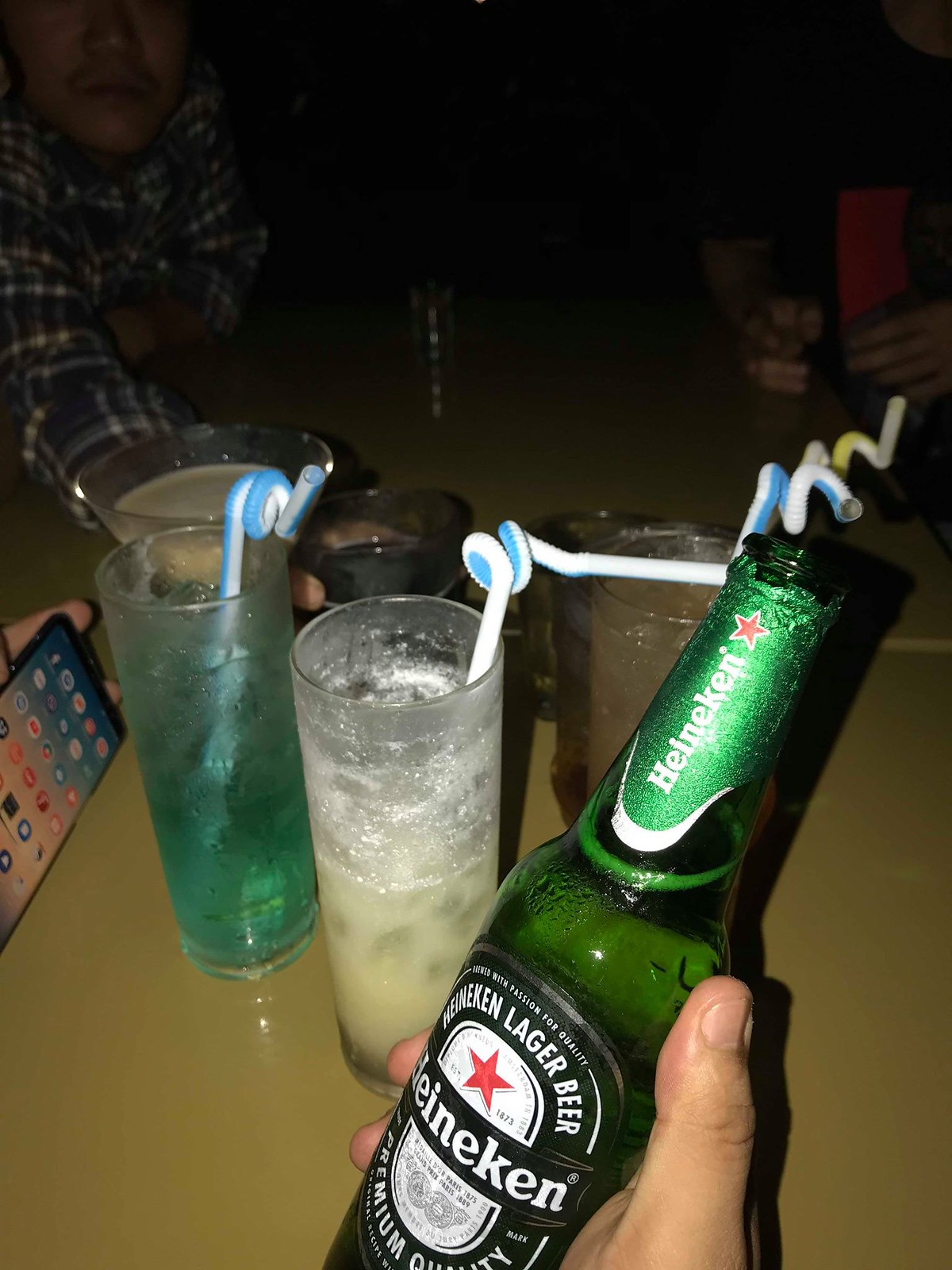In the dimly lit atmosphere of a bar or club, a long table is partially visible, adorned with an array of drinks and objects that tell the story of a night out. In the foreground, a Caucasian or light-skinned hand holds a green Heineken bottle, prominently displaying the iconic Heineken Lager Beer label with its white text and red star against a black background. The bottle, still containing some liquid, stands in contrast to the several empty tall narrow glasses around it. 

These glasses, each housing colorful, twirly straws— one blue with white stripes and the other white with blue stripes— hold remnants of mixed drinks: a cloudy white beverage and a clear green one. A phone rests at the bottom left corner of the image, near the hand holding the Heineken bottle. 

In the background, two individuals are seated at the same table. On the left, a man wearing a blue and white plaid long-sleeved shirt is partially seen with his hand on a cup. On the right, only the arms of another person in a black short-sleeved shirt are visible, resting on the table, creating a dynamic yet incomplete snapshot of an evening gathering.